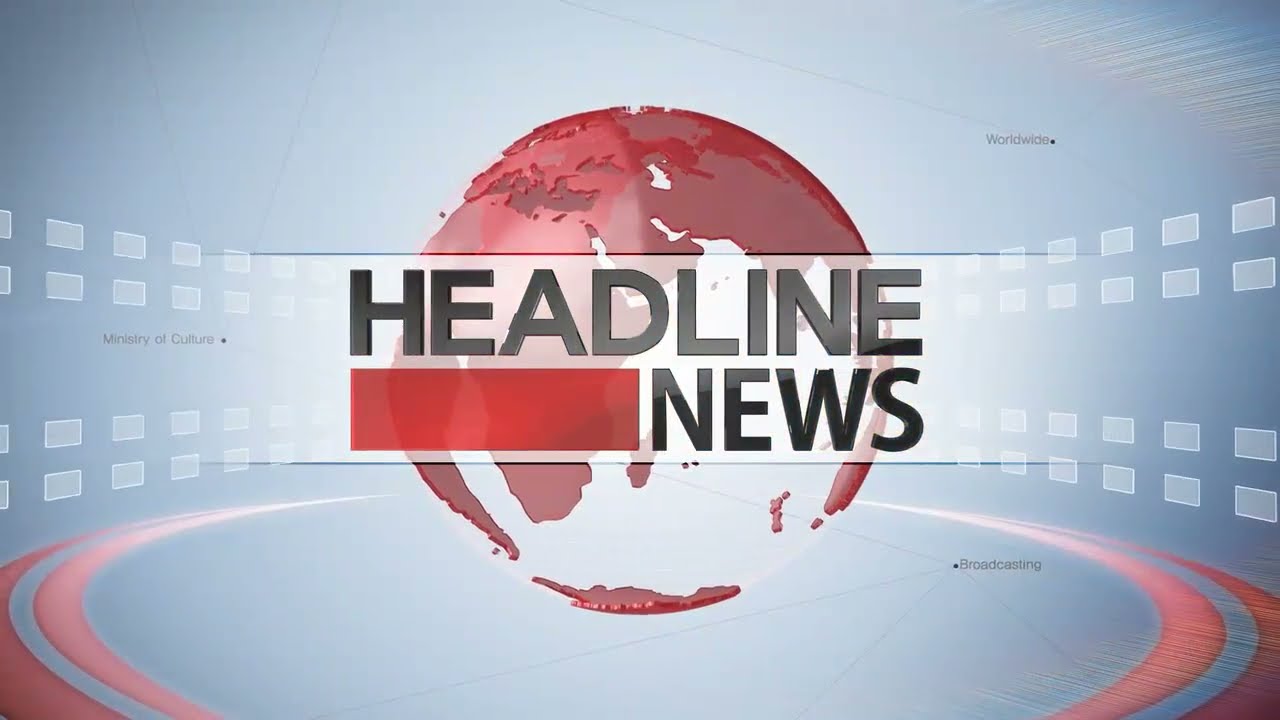In this detailed photograph, which appears to be a screenshot of a news broadcast, a news anchor of Asian descent is prominently featured at the center of the image. He has short black hair and is dressed in a black suit paired with a white collared dress shirt and a black tie, adorned with a yellow ribbon on his lapel. Holding a microphone, he addresses the camera. The lower third of the screen displays a white rectangular banner with a red stripe at the bottom. The banner reads "A Nation Mourns" in black letters, and to the left, columns list the numbers "Rescued 174," "Missing 131," and "Dead 171" in white text on a red background.

The background reveals a bustling newsroom setting filled with several TV screens mounted on the wall and various people working at cubicles. A significant feature of the environment is a red sign descending from the ceiling with white text that says "Arirang News," with "Arirang" written in a stylized cursive font. The dominant colors in the room are a red-and-white motif, though the back wall appears to be a blurry white or bluish hue, potentially due to lighting. Additionally, a woman with brown hair tied up and wearing glasses can be seen in the bottom right corner with her back facing the camera.